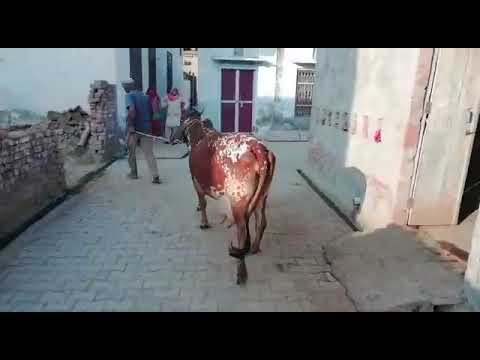The photo captures an outdoor scene featuring an old cobblestone walkway framed by crumbling brick walls and aged stone buildings. A man, dressed in a blue short-sleeved shirt and beige pants, is pulling a rope attached to a bovine animal, possibly a cow. Both the man and the cow are facing away from the camera. The man, who appears to have dark skin and is wearing a light round cap, is guiding the skinny, brown cow with scattered white spots along the brick-paved road. On the right side, a concrete ramp leads to an open doorway in a white, slightly dirty stone building. Behind them, there’s another perpendicular walkway bordered by buildings with white walls, burgundy doors, and gated windows. The sun is casting shadows, amplifying the worn, rustic charm of the surroundings.